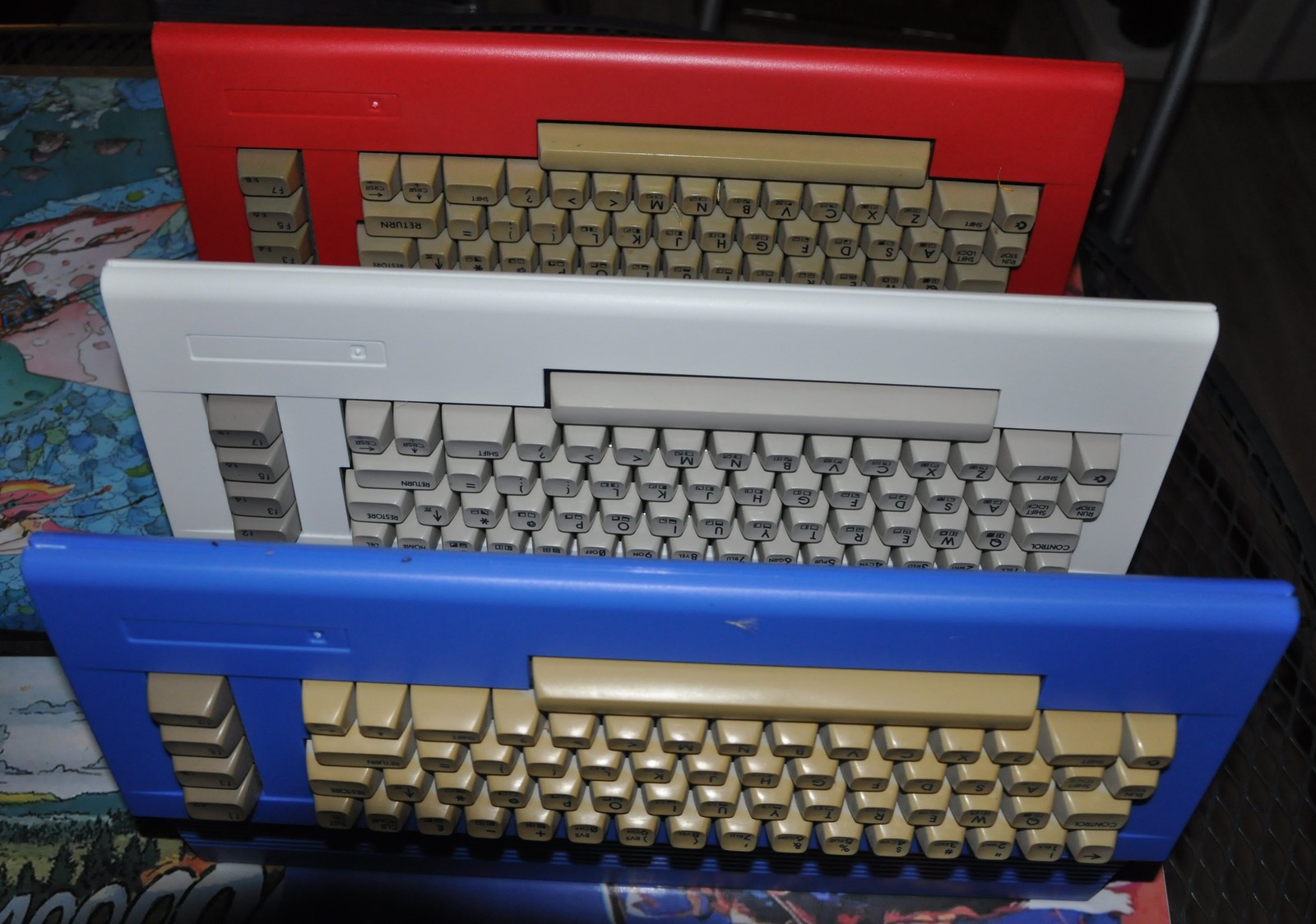The image depicts a vibrant and colorful scene with a background that resembles a hand-drawn forest, complete with trees, grass, and clouds. The foreground showcases three computer keyboards stacked vertically, each turned upside down with their spacebars pointing upwards. The top keyboard is red and adorned with golden keys, the middle one is white with gray keys, and the bottom keyboard is bright blue with golden keys. The keyboards appear to be made of plastic with high molded keys, and their frames are also plastic. To the left of the keyboards, there is a cloth featuring a complex blue and pink design, likely pictorial in nature, with some possible numeric elements at the bottom. The left-hand side of the image includes a slightly reflective black area, with a noticeable line and more reflections in the top left corner.